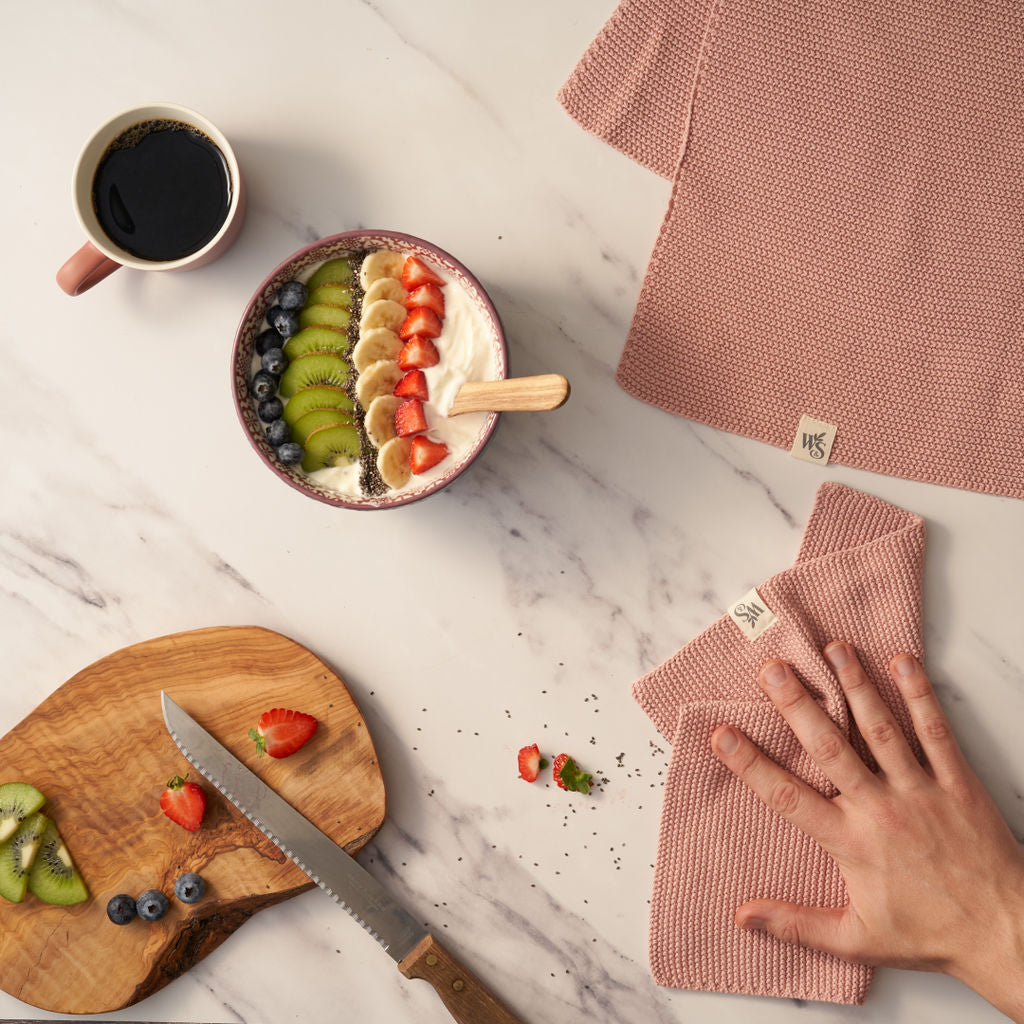An overhead view captures an inviting kitchen scene centered around a wooden counter or table. At the heart of the image is a bowl of creamy white yogurt, elegantly garnished with meticulous rows of vibrant fruits: deep blue blueberries, luscious green kiwi slices, perfectly rounded banana pieces, and juicy red strawberries, all arranged symmetrically. A wooden spoon stands ready in the bowl, suggesting an imminent, delightful blend of flavors. To the right of the bowl, a wooden cutting board with a serrated knife reveals the ongoing preparation, dotted with freshly sliced strawberries, blueberries, and kiwis. In the upper left corner, a comforting cup of rich, dark coffee adds warmth to the scene, hinting at a cozy breakfast or snack in progress.